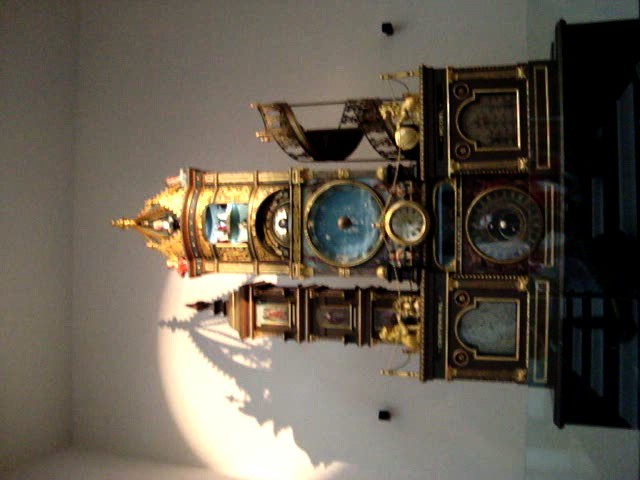This photograph features a detailed model of a mini clock tower inside a building. The image is oriented sideways, causing the top of the model to point to the left instead of upwards. The clock tower model stands on a black dresser against a light cream-colored wall. Sunlight streams through a window, casting a bright illumination predominantly on the top of the model, which is primarily golden in color interspersed with blue details. The tower has a central ring in gold, and there are light blue elements visible within it. The structure also includes smaller, darker towers on either side, one featuring a spiral design resembling a staircase. The intricate model exhibits elements suggesting an 18th-century village setting, with mixed shades of brown and red incorporated into its design.